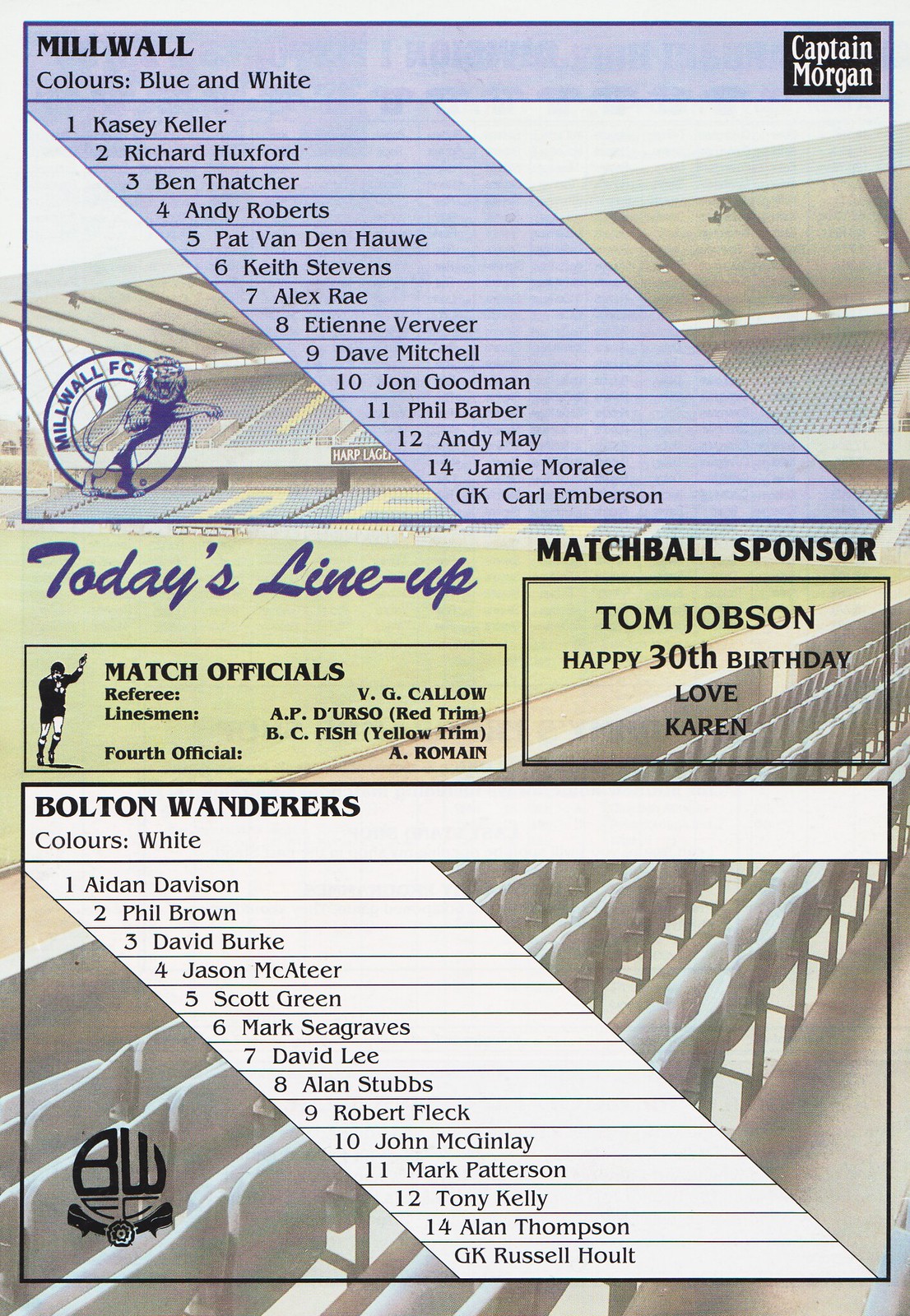The image showcases a scanned page from a match day magazine for a soccer game between Millwall and Bolton Wanderers. The background features an empty sports stadium. On the top section, encased within a blue-bordered box, it lists the Millwall team lineup in blue and white colors: 1. Casey Keller, 2. Richard Huxford, 3. Ben Thatcher, 4. Andy Roberts, 5. Pat Van De Howe, 6. Keith Stevens, 7. Alex Ray, 8. Etienne Verveer, 9. Dave Mitchell, 10. John Goodman, 11. Phil Barber, 12. Andy May, 14. Jamie Morelli, and goalkeeper Carl Emberson. 

The central part of the page provides information about today's match officials, including referee VG Gallo and linesmen AP Durso (red trim) and BC Fish (yellow trim), along with the fourth official A. Romain. Additionally, there's a birthday note wishing Tom Jobson a "Happy 30th Birthday" from Karen, tied to the match ball sponsorship.

At the bottom, similarly structured, the section outlines the Bolton Wanderers team in white: 1. Aidan Davidson, 2. Phil Brown, 3. David Burke, 4. Jason McAteer, 5. Scott Green, 6. Mark Seagraves, 7. David Lee, 8. Alan Stubbs, 9. Robert Fleck, 10. John McGinley, 11. Mark Patterson, 12. Tony Kelly, 14. Alan Thompson, and goalkeeper Russell Holt. 

The upper right corner of the page is marked with a distinctive “Captain Morgan” logo, indicating sponsorship or branding.